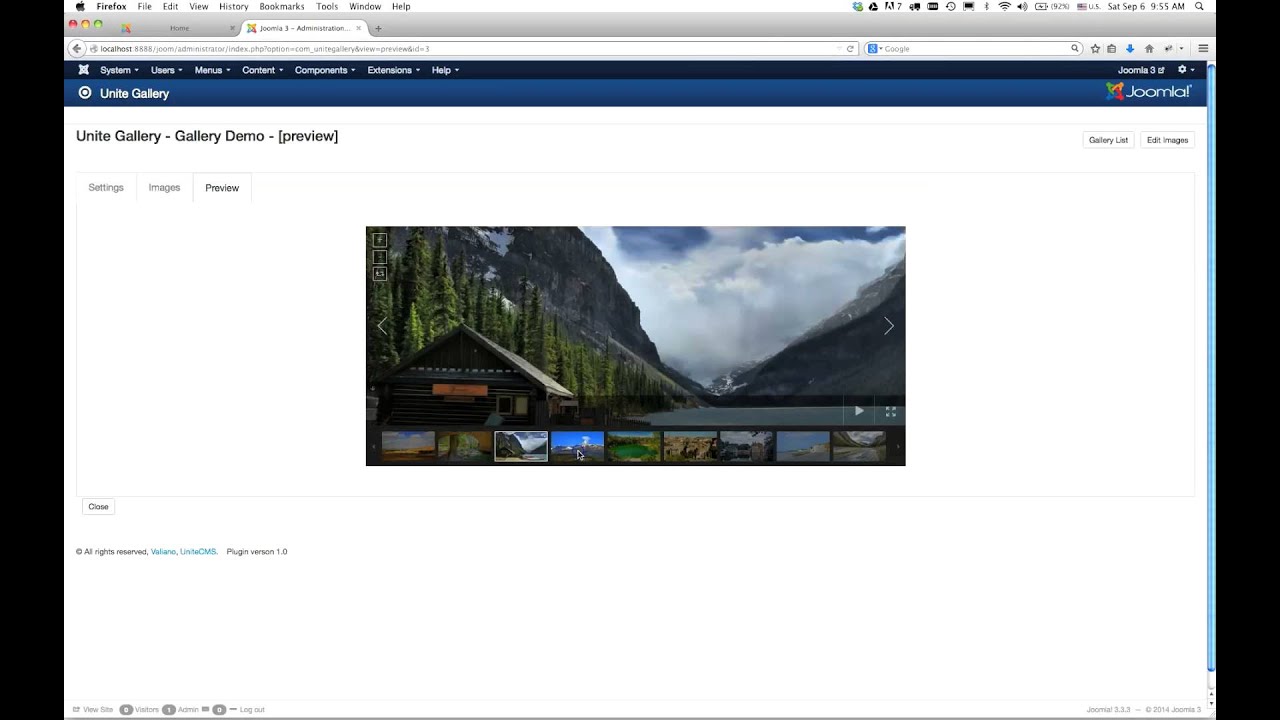This image showcases a demo of the Unite Gallery interface, highlighting various features for photo display and user interaction. The focal point of the image is a picturesque cabin situated at the front left, set against a backdrop of lush trees on steep bluffs that reach skyward, creating a majestic valley scene. A serene river or lake runs through the middle, flanked by shorter, gently sloping areas on the right. Puffy clouds dot the sky, adding to the tranquil ambiance.

The gallery interface is active, displaying one of the slides, with several thumbnail images below that can be clicked to enlarge different photos. At the top of the screen, familiar browser buttons are visible, indicating the use of an Apple device with Firefox open. It showcases the standard menu options like File, Edit, View, History, Bookmarks, and more, alongside a single open tab.

Below the address bar—which is currently set to the Unite Gallery website—there is an option for a Google search. The header "Unite Gallery" is prominently displayed in white against a blue background, credited to Joomla (J-o-o-m-l-a). The section also announces this as a "Unite Gallery - Gallery Demo Preview" with buttons for "Gallery List" and "Edit Images" available on the far right. At the very bottom, the footer notes "All rights reserved" and specifies the plug-in version (1.0).

Overall, this detailed depiction not only captures the aesthetic elements of the displayed image but also the functional aspects of the gallery demo interface.